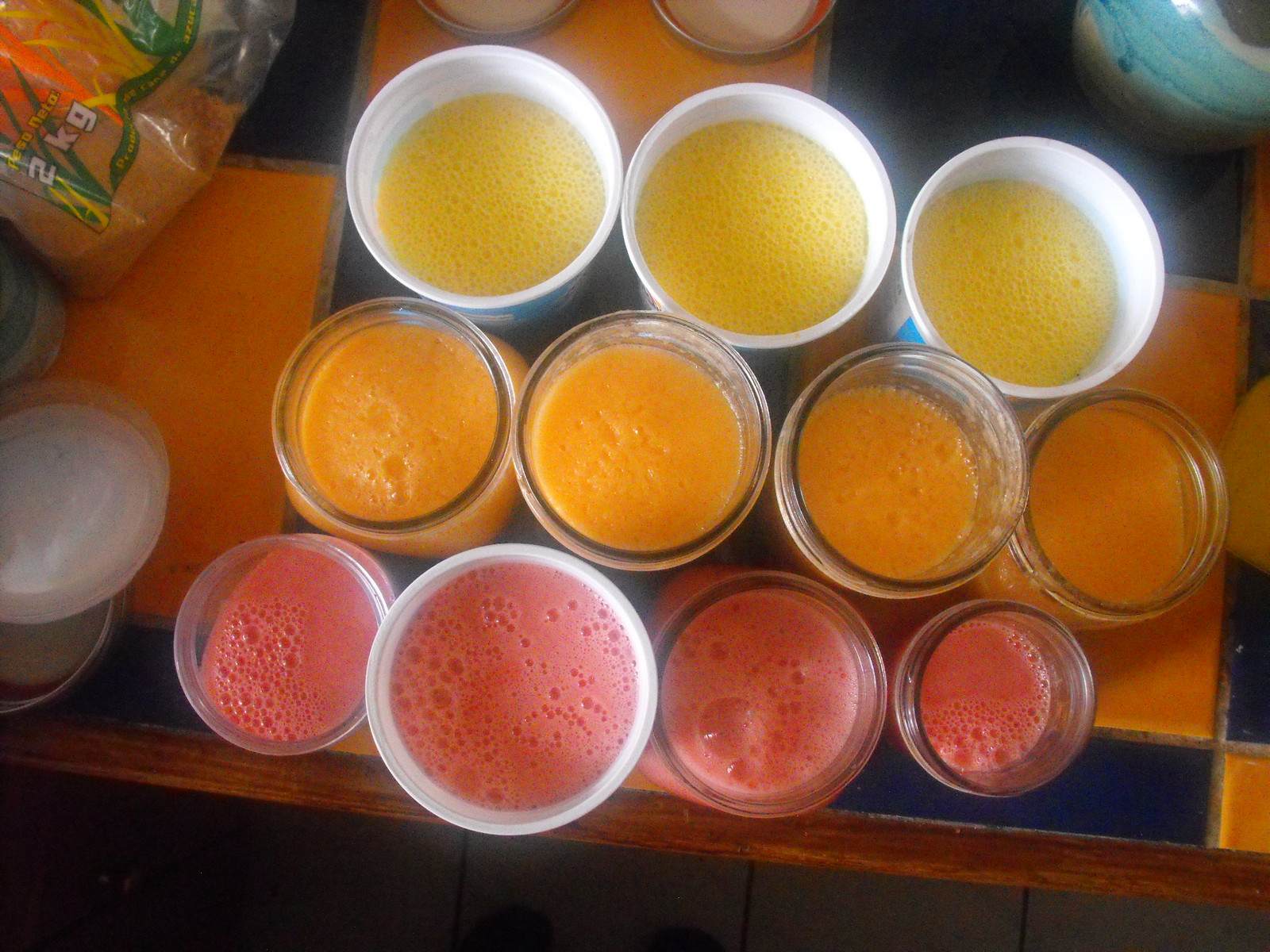This detailed top-down photograph captures three rows of 11 frothy, bubbly juice beverages arranged neatly on a ceramic-tiled tabletop. The tabletop features a striking checkered pattern of alternating black and orange tiles. 

In the top row, there are three white paper cups, each filled with frothy yellow juice, likely pineapple-flavored agua fresca. The middle row consists of four clear glass cups, each containing bubbly orange juice that might be cantaloupe-flavored. The bottom row has three more glass cups and one white paper cup, all filled with a light red, foamy liquid, probably watermelon-flavored. 

The tabletop has a wooden trim, adding a rustic charm, and the surroundings include a plastic bag marked with "two kilograms" in the upper left corner and the edges of someone's shoes faintly visible at the bottom. This composition suggests an inviting, vibrant scene possibly set in a casual restaurant.